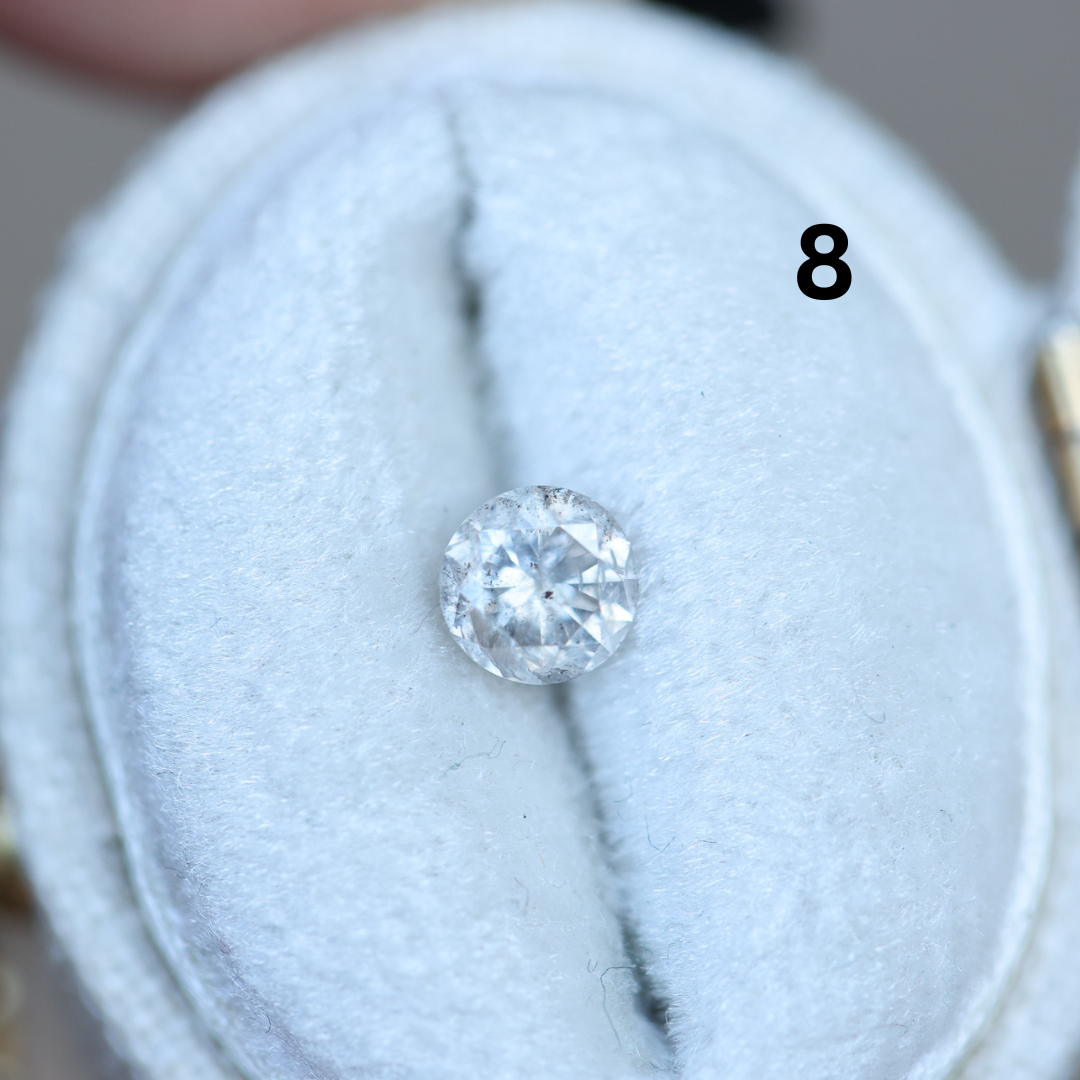This image showcases a large, solitary diamond, prominently set against a white, oval-shaped background that features a central dark crease. This oval backdrop, resembling a soft pillow or felt fabric, appears to be part of a display or jewelry holder. The diamond, potentially a princess cut due to its bright and shiny appearance, is circular and markedly clean, despite some suggestions otherwise. Bold black letters display the number 8 on the background, likely indicating the diamond's catalog or identification number. The entire scene seems to be framed or held within a square setting, possibly part of a jewelry box or a hinged lid mechanism, as suggested by hints of brass or gold visible around the edges. Touches of a gray background and what might be part of a human hand provide additional context to this photograph, which captures an elegant yet simple presentation of a standalone, dazzling gemstone.